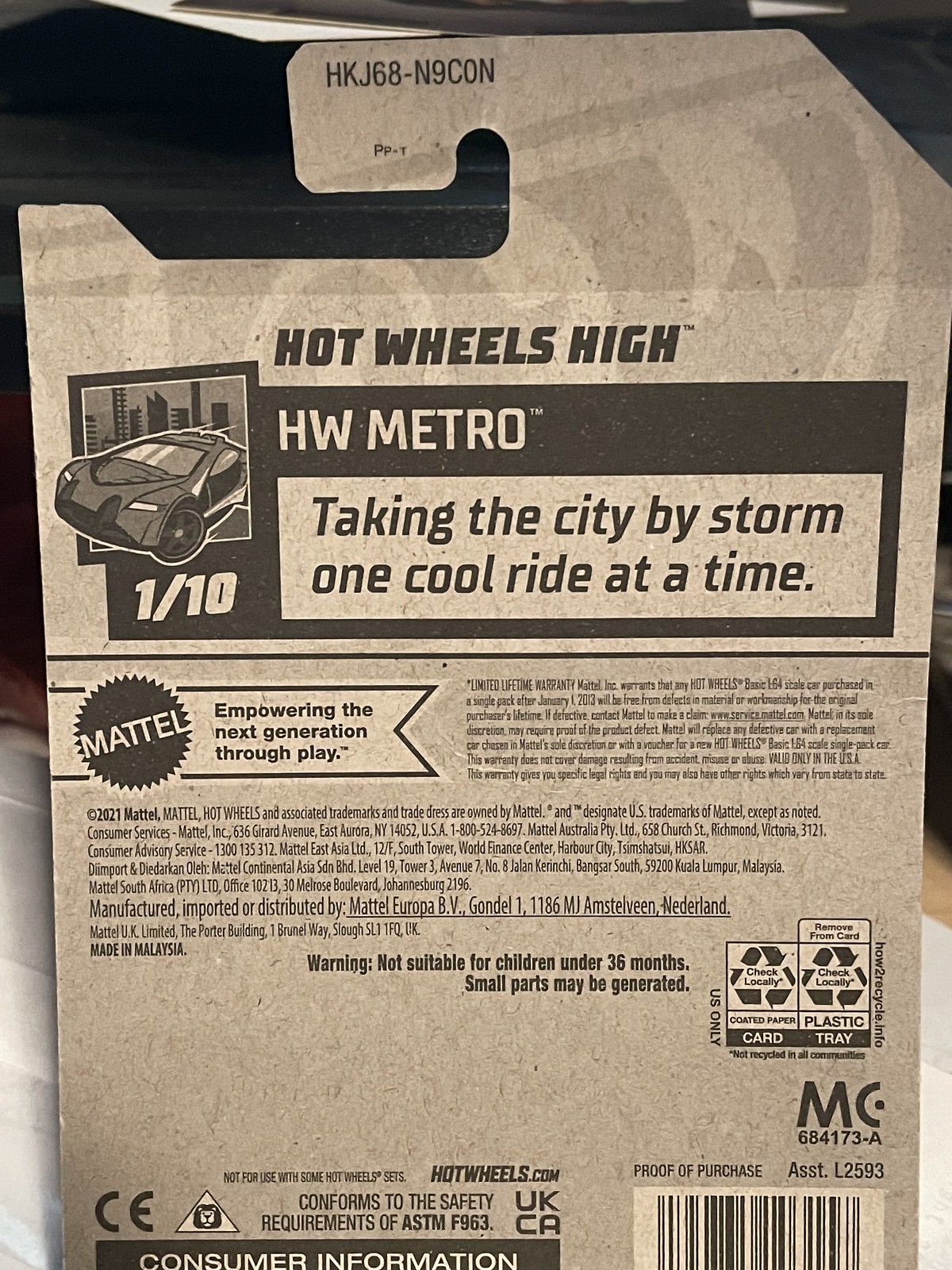The image depicts the back of a Hot Wheels package. At the top, bold text reads "Hot Wheels High" and "HW Metro," followed by the slogan in italics: "Taking the city by storm, one cool ride at a time." On the left, there's an image of a sports car emerging from a box with a cityscape in the background, labelled "1/10" in white letters. Beneath this, the Mattel logo is prominently displayed with the mission statement, "Empowering the next generation through play." Small black text fills the space with various consumer details, and the bottom right features a barcode, indicating proof of purchase, and details about the recyclable nature of the packaging materials. The bottom left contains a consumer information section and a warning: "Not suitable for children under 36 months, small parts may be generated." The cardboard has a gray color with dark lettering scattered throughout.